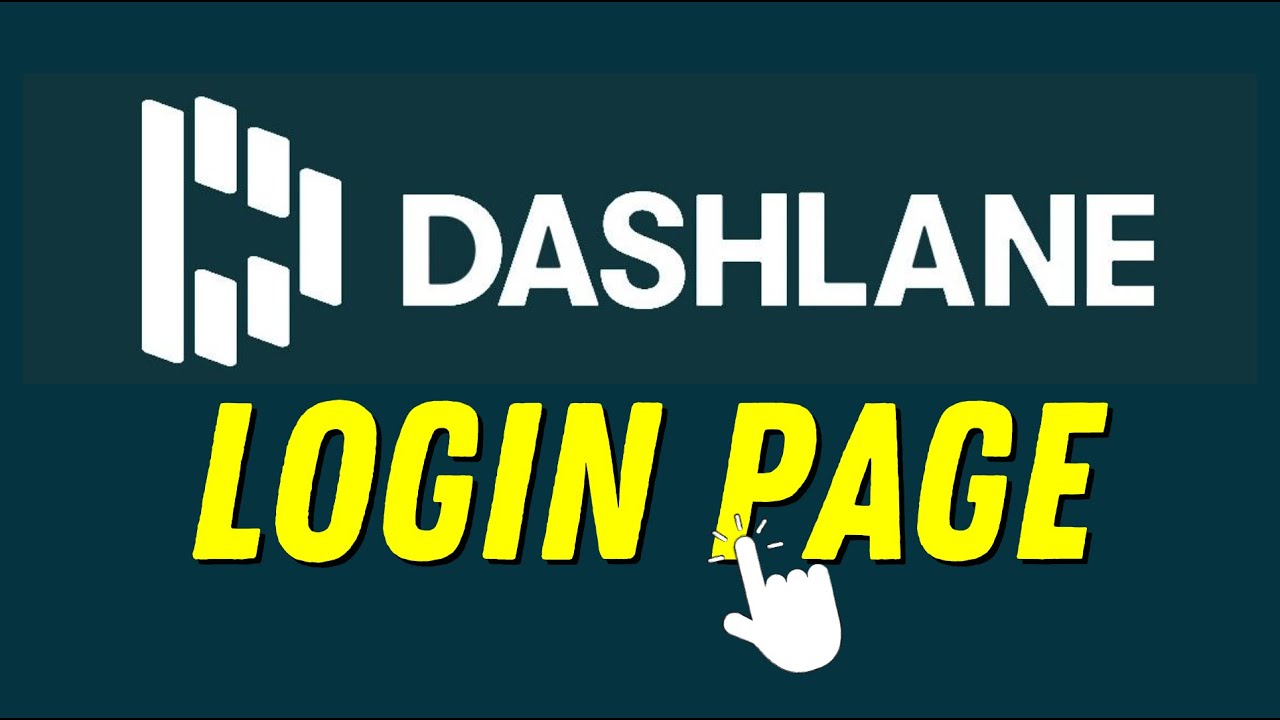This is a detailed and cleaned-up caption for the described image:

"This banner ad features a large, slightly rectangular layout with a deep bluish-green background. At the top, in bold white lettering, the brand name 'Dashlane' is prominently displayed, accompanied by the Dashlane logo to its left. Below the brand name, 'Login Page' is written in vibrant yellow text. A white cartoon glove finger icon is illustrated tapping on the 'P' of 'Login Page,' with motion lines indicating the tapping action. This visually engaging banner suggests that clicking or tapping on the ad will direct users to the Dashlane website, where they can access the login page or create a new account. The overall design combines striking colors and clear branding to effectively capture attention and convey its purpose."